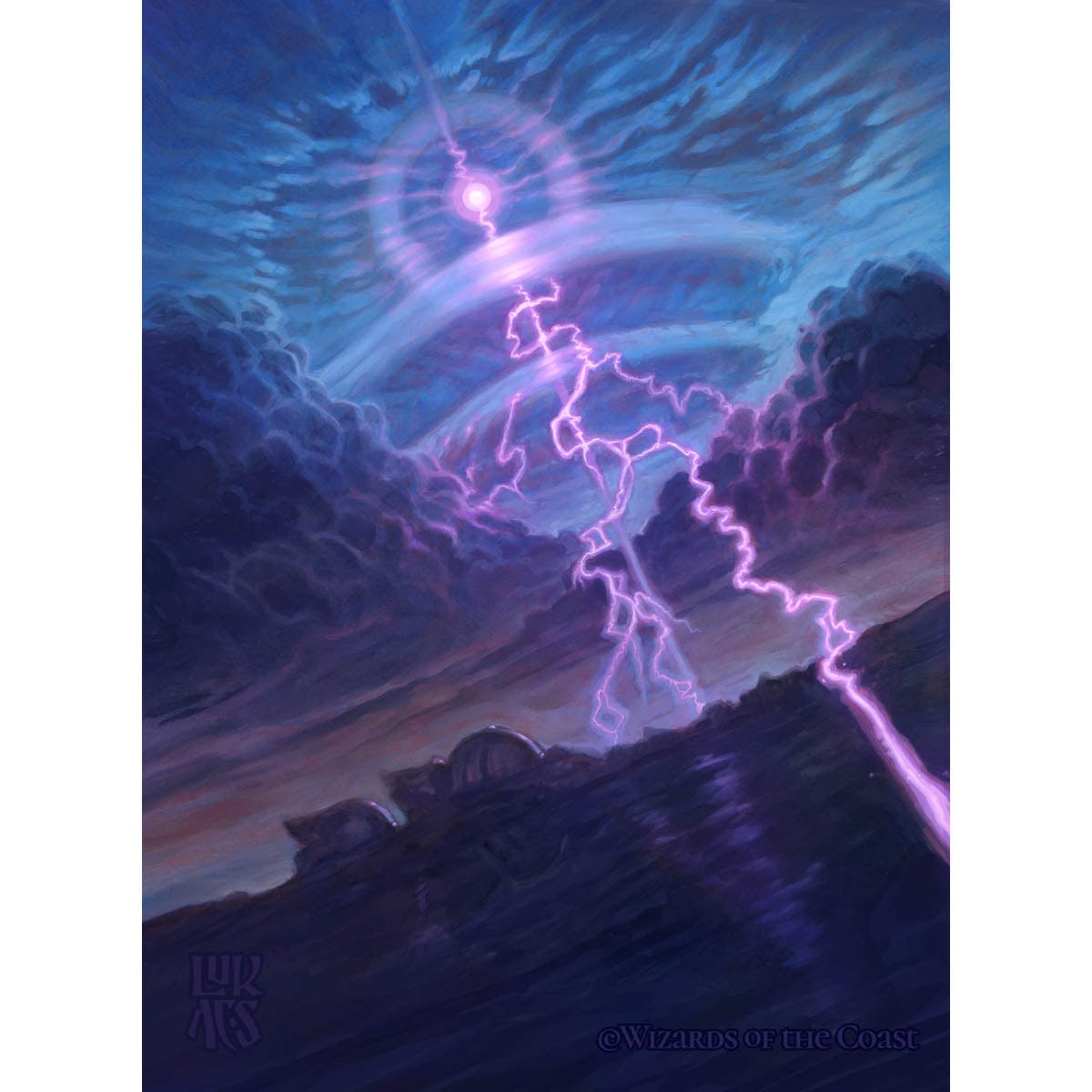The vertical rectangular image appears to be a detailed fantasy illustration prominently featuring dramatic lighting effects and surreal landscapes. In the sky, there is a significant blue circle with a halo effect, suggesting an intense focal point of light, surrounded by swirling clouds, resembling a vortex. Below this circle is a smaller, cone-shaped form acting like a conduit for the pink, squiggly lines of energy emanating upward from the ground. These pink lines converge at the base of the blue cone and emit blue waves that spread outwards from its top.

Beneath this sky-bound spectacle is a surreal terrain featuring dark, tipped ground with a sideways orientation, possibly suggesting a disorienting perspective. The ground looks like dark water or desert, and includes mesas and cliffs in the background. There are also vivid, chaotic elements such as pink lightning bolts and scattered purple electrical discharges, contributing to a sense of dynamic, otherworldly chaos. The combination of dark and bright colors, twisted earth, and dramatic sky make the image appear intensely imaginative and cosmic. Notably, the artwork is branded with a watermark in the lower right corner, indicating it is produced by Wizards of the Coast.